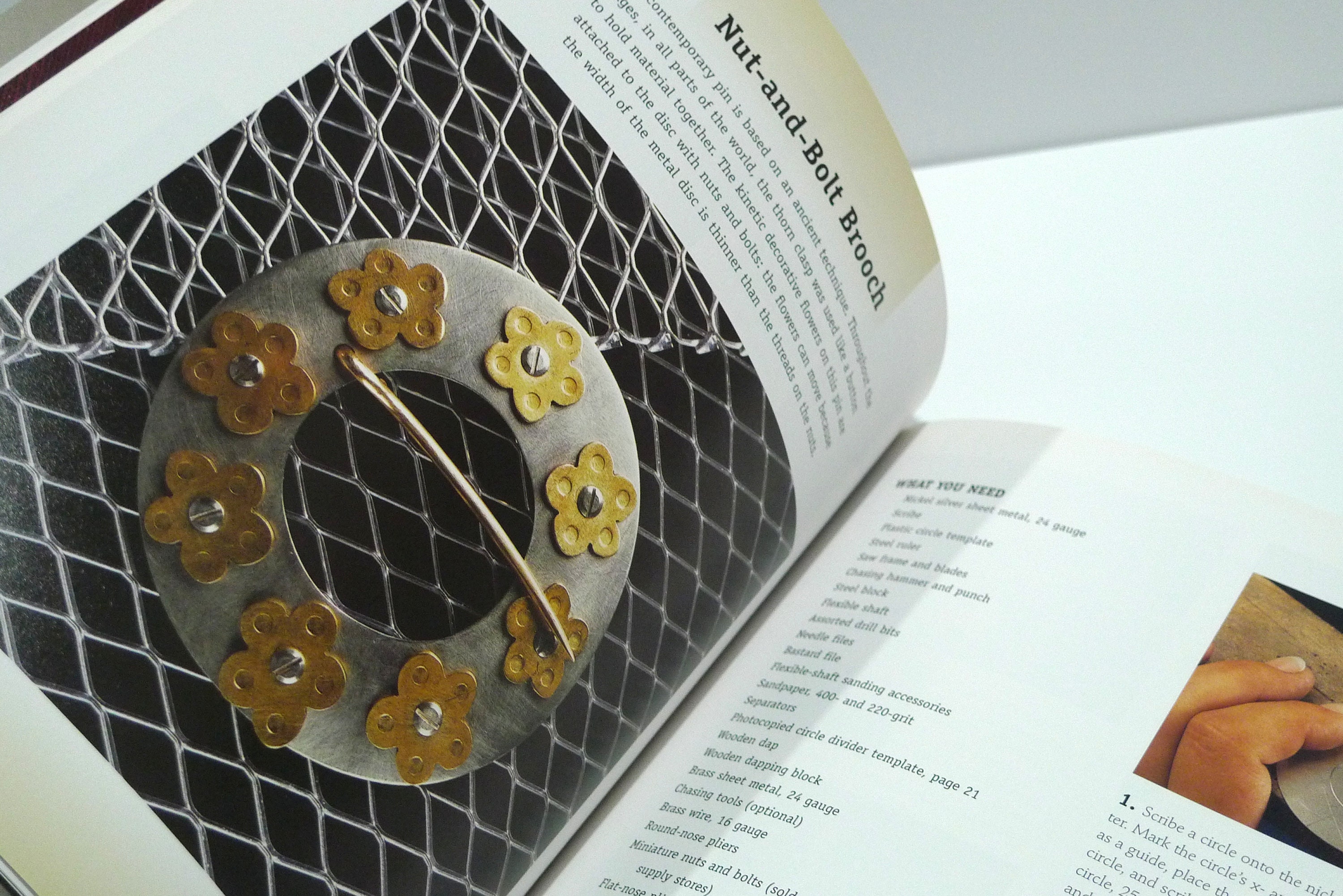The photo captures an open book placed diagonally near the center and bottom of the image. The book's white pages feature black text and are highlighted against a white and grey backdrop in the top right corner. Featured prominently on the page is a photograph of a circular metal brooch with intricate, gold-plated floral patterns arranged in a wreath-like formation around a central needle or pin. The brooch rests on a grey wire mesh background. On the left page, a headline reads "Not in Bold Brooch," with a descriptive paragraph below. The right page contains a list under the title "What you need," detailing materials and instructions for crafting the brooch. The setting harmoniously blends elements of jewelry and books, with both the book and the underlying tabletop in shades of white.